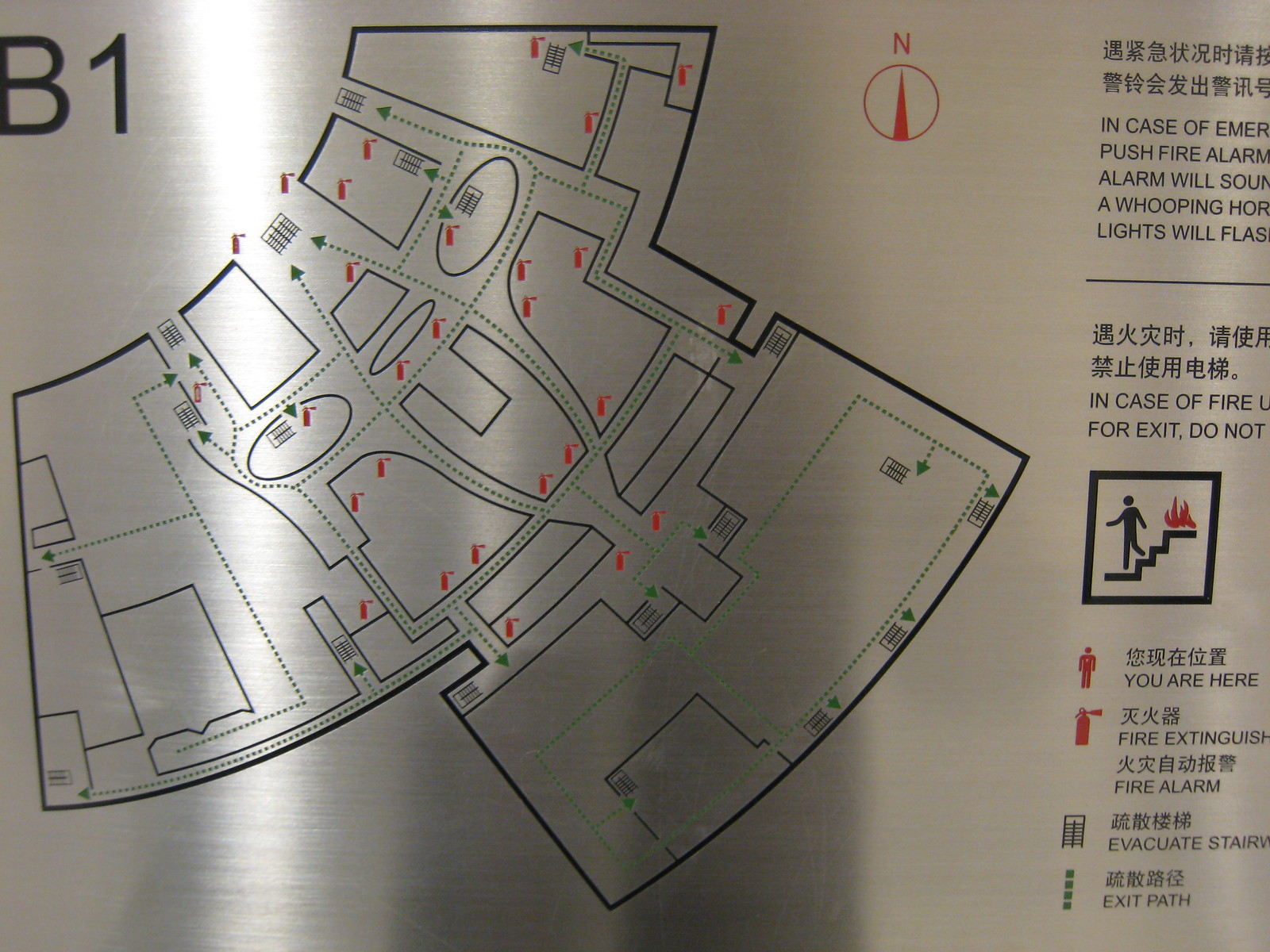The photograph depicts an emergency evacuation map, likely fixed to a wall, detailing the layout of a building's floor, identified at the top left as "B1." The map prominently features red indicators for fire extinguisher locations and uses a red human figure to denote the viewer's current position with the label "You Are Here." A detailed compass in the top left indicates the direction "North," and to its right, Chinese characters are present with an English translation below them, instructing: "In case of emergency push fire alarm. Alarm will sound a whooping horn, lights will flash." Although the full text is partially obscured, its essence is conveyed.

The image is mostly in black and white, except for the bright red icons indicating fire-related elements. The map legend in the bottom right includes a green dot representing the exit path and an icon for the evacuation stairway, marked clearly next to a stairwell diagram. Additional keys explain various other symbols used throughout the map, such as fire extinguishers and evacuation routes, providing clear guidance on how to exit the building safely in an emergency.